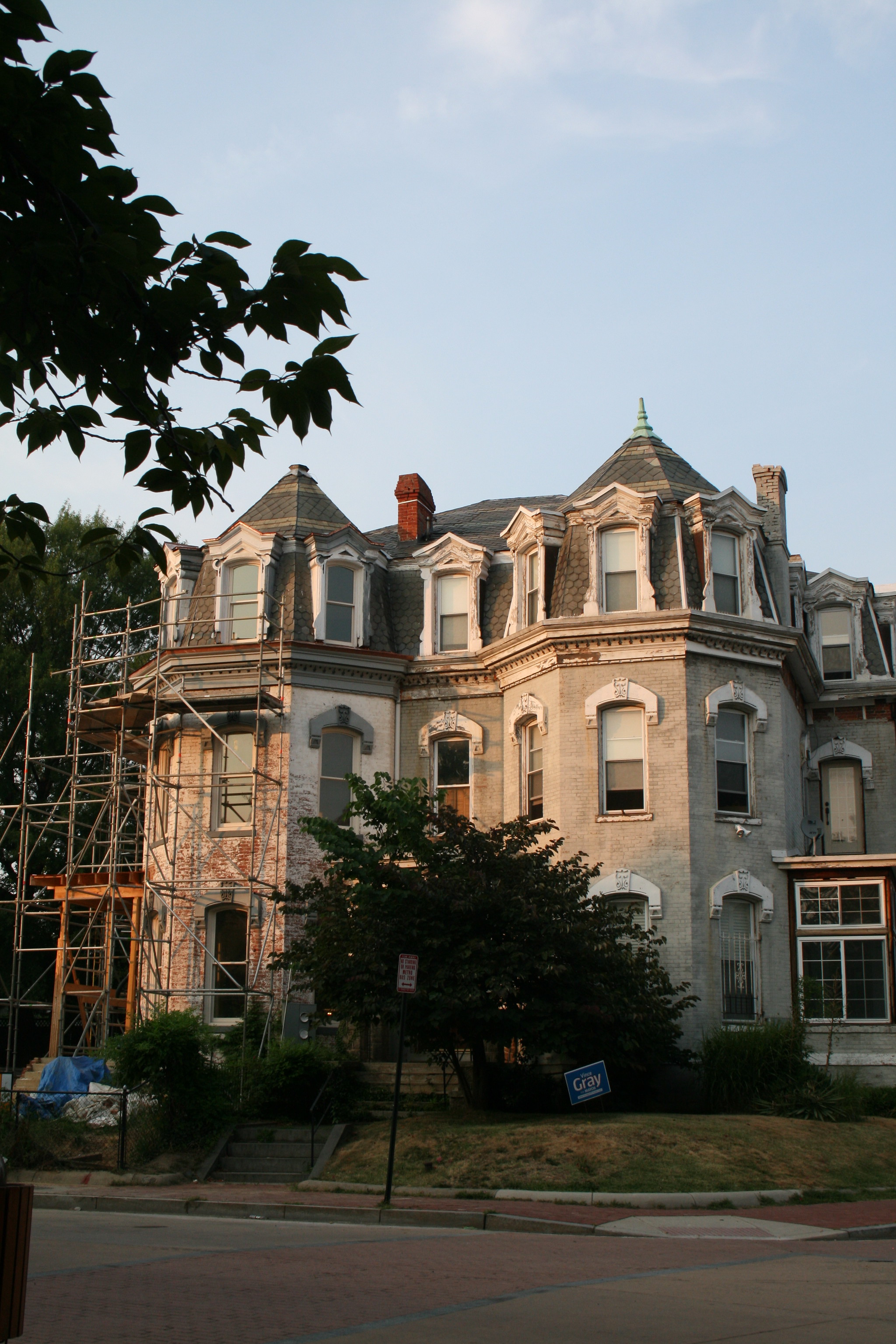The image depicts a three-story, older-style castle-like house undergoing renovation. The house, which features a combination of Victorian and Federalist architectural elements, is built from red brick and has been painted white, though red bricks are visible through areas where the paint is being removed. The left side of the house is heavily scaffolded, with a blue tarp at the base, indicating significant restoration work. The roof is gray and shingled, adorned with ornate windows that circle around cylindrical tower sections attached to the house. A prominent red brick chimney complements the structure. On the right side, there is a small enclosed entranceway with numerous windows and red walls.

The house sits atop a slight hill, accessed by two sets of concrete stairs. In the yard, there is a slightly askew blue political sign with unreadable yellow letters. The surrounding area includes a no parking sign, a red sidewalk with a white slope leading down to the street, which also has red brickwork in the center. A large tree partially obstructs the view of the front door and the lower level, with additional tree branches visible from the top edges of the image, suggesting the photograph is taken at street level. The clear sky, with a few clouds, and the lighting hint that the photograph was taken either early in the morning or late in the afternoon.